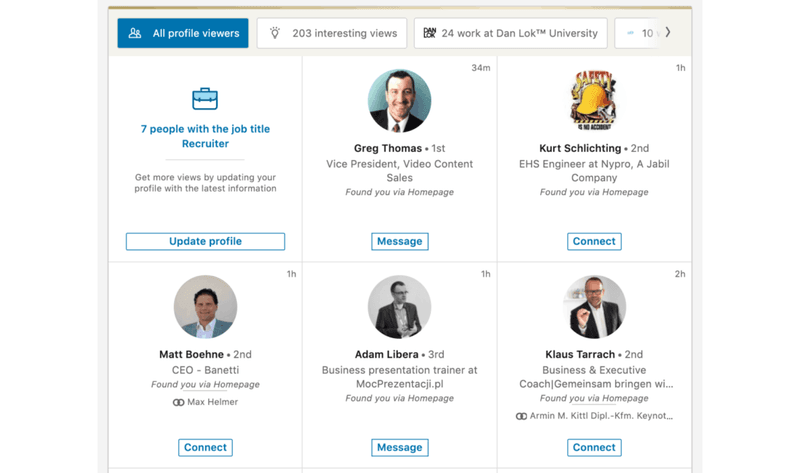This is a detailed caption for an image showing profile users on a recruiting website. The screenshot features a structured layout with three profiles across and two down. At the top, a blue button labeled "All Profile Viewers" and "203 interesting views" are prominently displayed. The first profile, located in the upper left, shows a briefcase icon and the text "7 people with job title recruiter" in blue. A male profile image of Greg Thomas is shown; he is looking forward and wearing a suit. His title is "First Vice President in Video Content Sales," and it indicates he found you via the homepage. There is also a button to message him.

To the right of Greg's profile is Kurt Schlittening, an engineer, illustrated with a hard hat logo above his profile image. There is an option to connect with him. On the second line, the first profile belongs to Matt Bone, CEO of Benetti, with an option to connect. Next to him is Adam Libera, a business presentation trainer at macpresenteaxi.pl, shown in a black and white picture. There is an option to message him. The final profile on the right is Klaus Turok, whose photo depicts him with a quirky look, facing forward with his hand held up in an exaggerated pose. He is listed as a business and executive coach with an option to connect. This overall layout suggests a recruiting website.